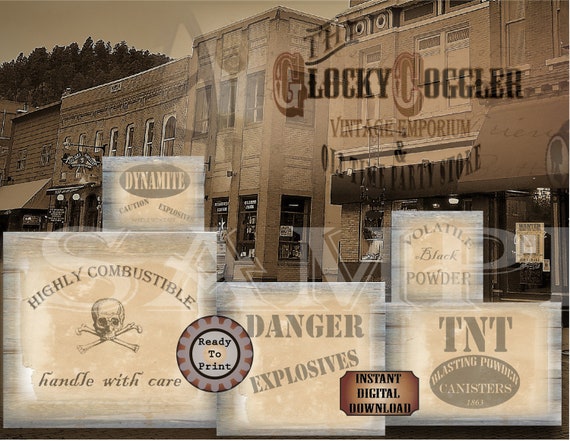This image presents a distinctive blend of historical and digital elements in a visually striking collage. The background features an old-style, two-story downtown city scene, possibly a main street adorned with vintage buildings, some of which are fronted by trees. The photograph appears to be black and white with a subtle red tint, adding to its aged appearance.

Prominently superimposed on the top right-hand side of the image is the text "Glocky Cobbler Vintage Emporium and Old Time Party Store" written in an old Western font, evoking a sense of nostalgia. The bottom half of the image showcases a series of vintage-style labels and warnings. These include a variety of cautionary texts such as:
- "Highly Combustible, Handle with Care" accompanied by a skull and crossbones.
- "Dynamite, Caution Explosives", positioned above the highly combustible warning.
- "Danger Explosives" featured centrally among these labels.
- "TNT Blasting Powder Canisters, 1863" along with "Volatile Black Powder" on the right side.

Additionally, there are two modern digital icons superimposed, adding a dash of modernity to the vintage theme. One is a circular badge reading "Ready to Print" and another resembling a ticket stating "Instant Digital Download", both in color.

Together, these elements create a layered visual narrative that feels both historical and contemporaneously styled, encapsulating the spirit of vintage branding with a modern twist.